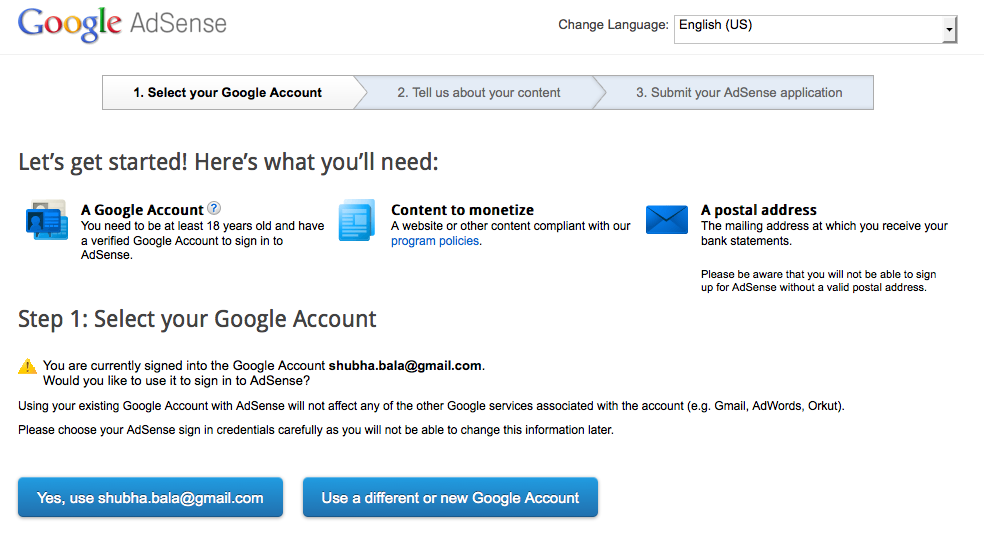This image showcases the landing page for Google AdSense account setup. At the very top, the page features the Google logo, the word "AdSense," and a drop-down menu for changing the language, which is currently set to English (US). 

Below the title, the page is divided into three main stages for setting up the account:

1. **Select your Google account** (currently selected)
2. **Tell us about your content**
3. **Submit your AdSense application**

The step-by-step guide begins with the current stage, "Select your Google account." The section starts with a welcoming prompt, "Let's get started," followed by a list of requirements:

1. **Google Account**: You need to be at least 18 years old and have a verified Google account to sign into AdSense.
2. **Content to Monetize**: A website or other content that complies with AdSense's program policies.
3. **Postal Address**: A valid mailing address where you receive your bank statements is essential for signing up.

Under the header "Step 1: Select your Google account," there's an alert message indicating that you are currently signed into the Google account Shubhabala@gmail.com and asking whether you would like to use it to sign into AdSense. Additionally, it reassures users that using their existing Google account for AdSense will not affect other Google services associated with the account, such as Gmail, AdWords, or Calendar.

There are two radio button options for the user:
- "Yes, use Shubhabala@gmail.com"
- "Use a different or new Google account"

The page is designed to guide users through the initial steps of setting up their AdSense account with clear instructions and options to proceed.